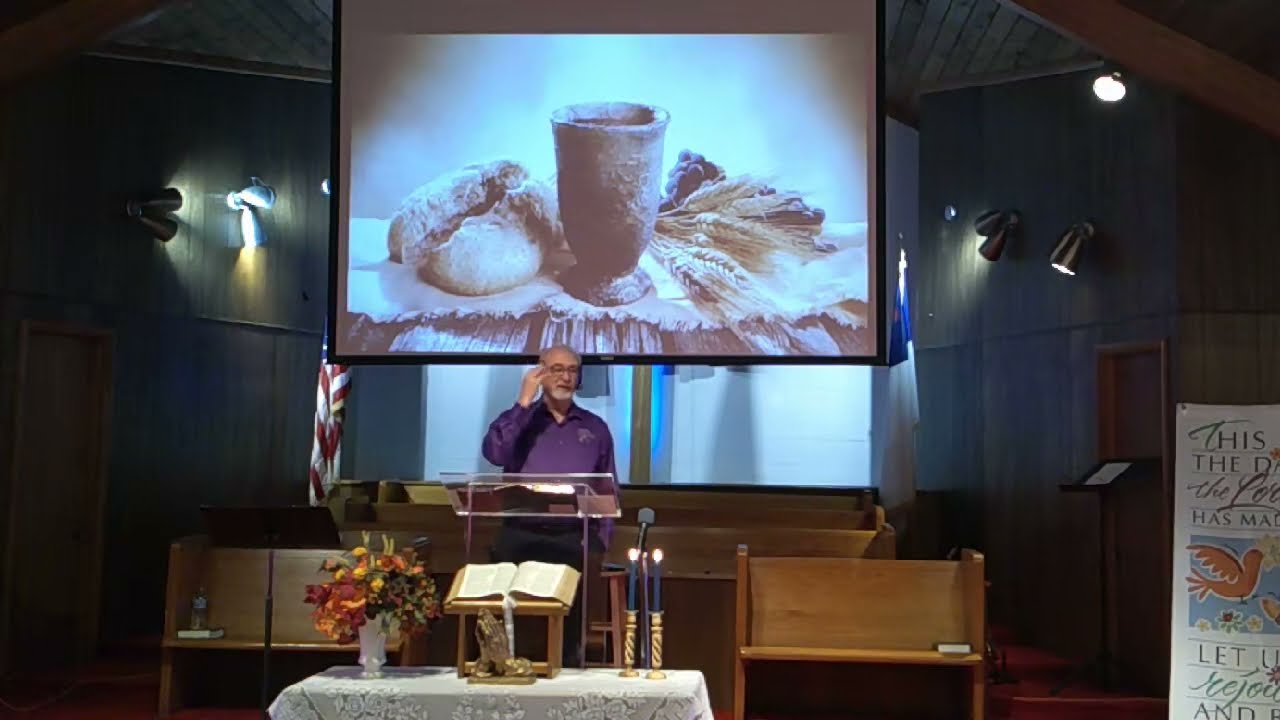In this screen grab of what appears to be a religious service filmed inside a church, an older man with grey hair and a beard stands at a clear glass or plastic podium. He is wearing a purple shirt and glasses, and he holds his right hand near his face, possibly interacting with an ear-fitted microphone or holding a clicker for the slideshow behind him. On the table in front of the podium lies an open Bible next to a bouquet of flowers. An American flag is positioned to his right. The backdrop features a projected image depicting a cup, a loaf of bread, and some wheat, likely symbolizing communion. Additionally, on the right lower corner of the projection screen, there is a sign reading, "This is the day the Lord has made, let us rejoice and be glad," accompanied by images of doves. Grey walls and a couple of lights accentuate the dramatic lighting of the scene, with pews visible in the background. The man appears to be the focal point, delivering a talk or sermon to an unseen audience.